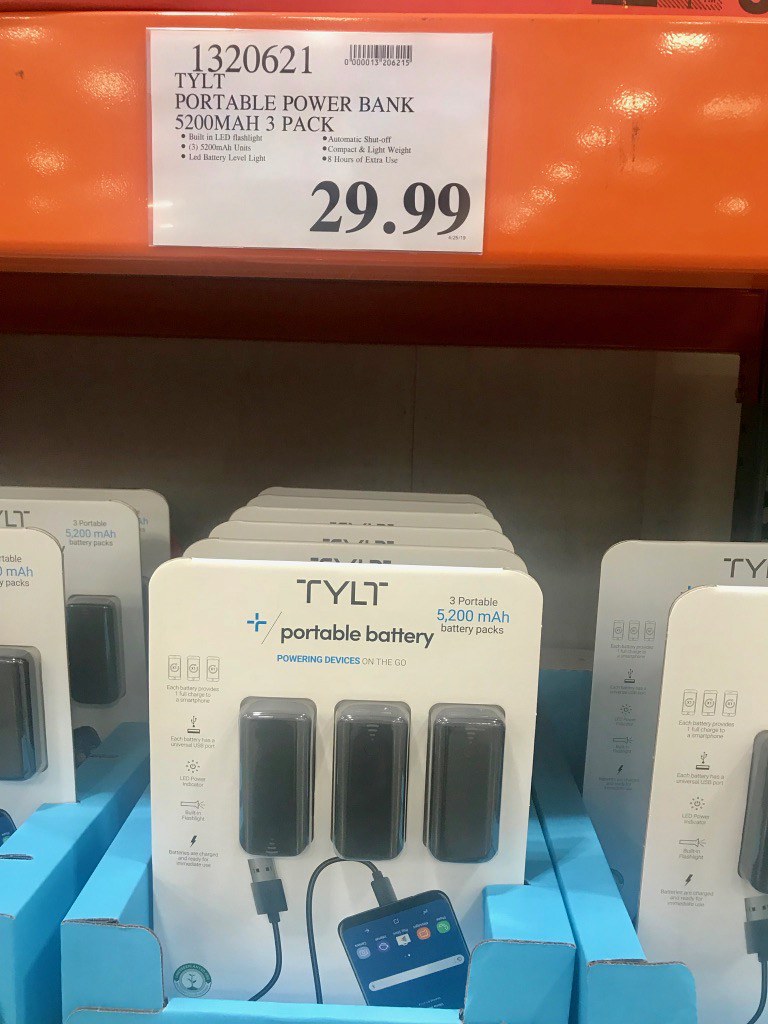This is an image from a store, likely a bulk retailer like Costco, featuring a shelf with an orange display and a white background. The display prominently showcases a white sign reading "1320621 TYLT Portable Power Bank 5200 mAh 3-Pack $29.99" in large letters. Below this sign, there are several blue cardboard holders containing the power banks, which are encased in clear, see-through plastic. Each package consists of three portable battery chargers, depicted as small black rectangles. The front of the packaging displays an image of a cell phone connected to one of the power banks via a wire, emphasizing the 5200 mAh capacity and the text "Power Devices." The overall setup has a structured alignment with multiple packages aligned front to back on the orange shelf.